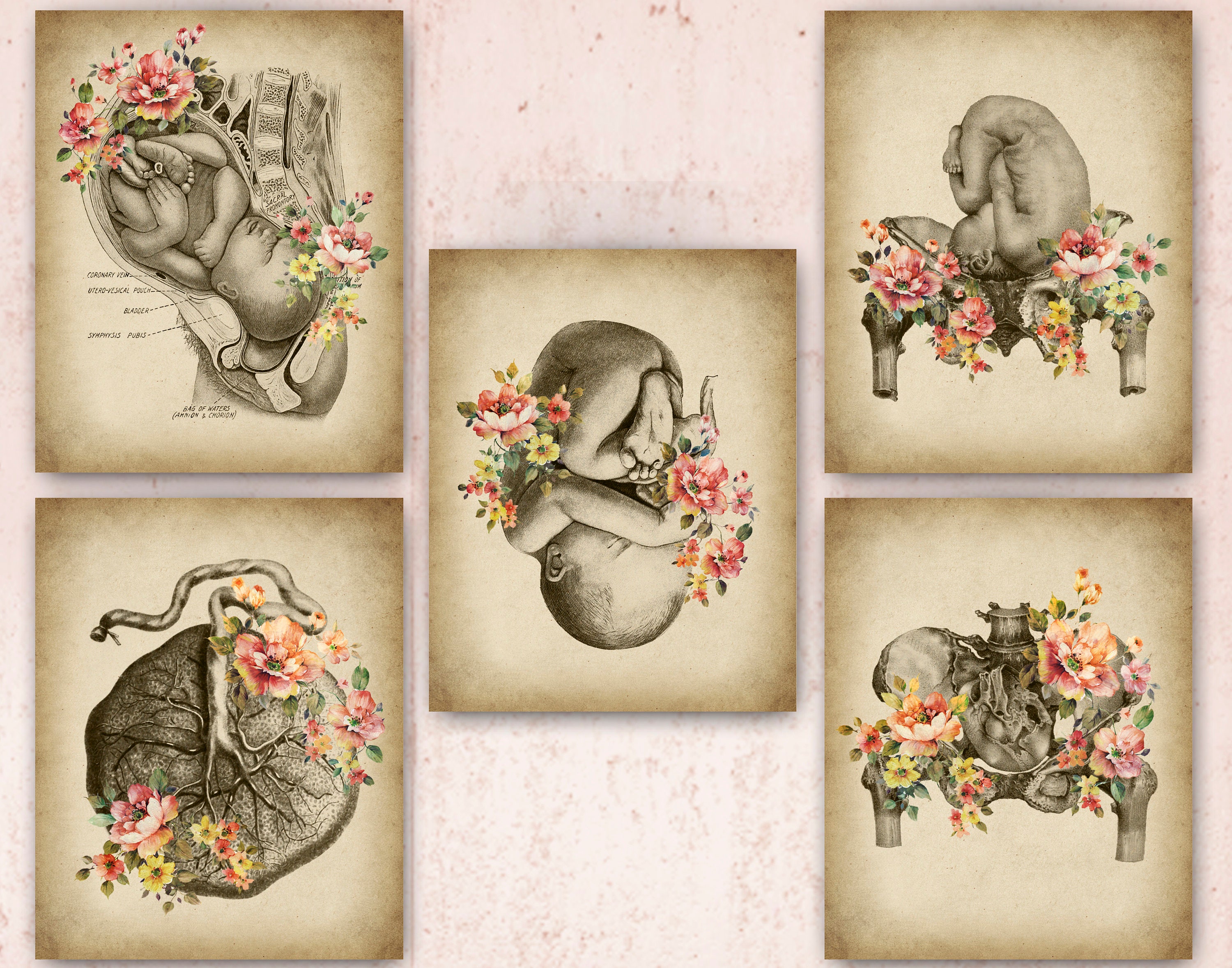The artwork features a series of five detailed illustrations depicting various stages of a baby's development in the womb, each set against a splotchy pink, light brown, and white background. The vertical panels, rendered in a faded beige hue, each present a unique perspective of the baby in utero.

1. The top left frame showcases a charcoal-style drawing of a nearly full-term baby curled up and upside down within the mother's womb. The baby’s head is near the bottom right of the frame, while its body arches toward the top left. Detailed anatomical sectioning of the woman's body is visible, adorned with pink flowers on the stomach area and a mix of pink and yellow flowers near the baby's head.

2. The bottom left frame presents a close-up of flesh with dark veins and an umbilical cord curving to the left. This segment is also highlighted with pink flowers on the bottom left and orange flowers on the top right.

3. The central frame features an upside-down baby without the surrounding womb, set amidst an array of pink flowers on both sides.

4. The top right frame depicts another upside-down baby nestled within a skeletal pelvis, with accompanying femurs on either side. Pink flowers embellish the left and right hip bones.

5. Finally, the bottom right frame mirrors the previous pelvic scene but includes an upside-down skull within the pelvis. This image is further decorated with pink flowers on the left and a combination of orange and pink flowers on the right.

Together, these frames intricately detail the stages of life in utero, enhanced with floral elements that add a touch of nature’s beauty to the developmental journey.